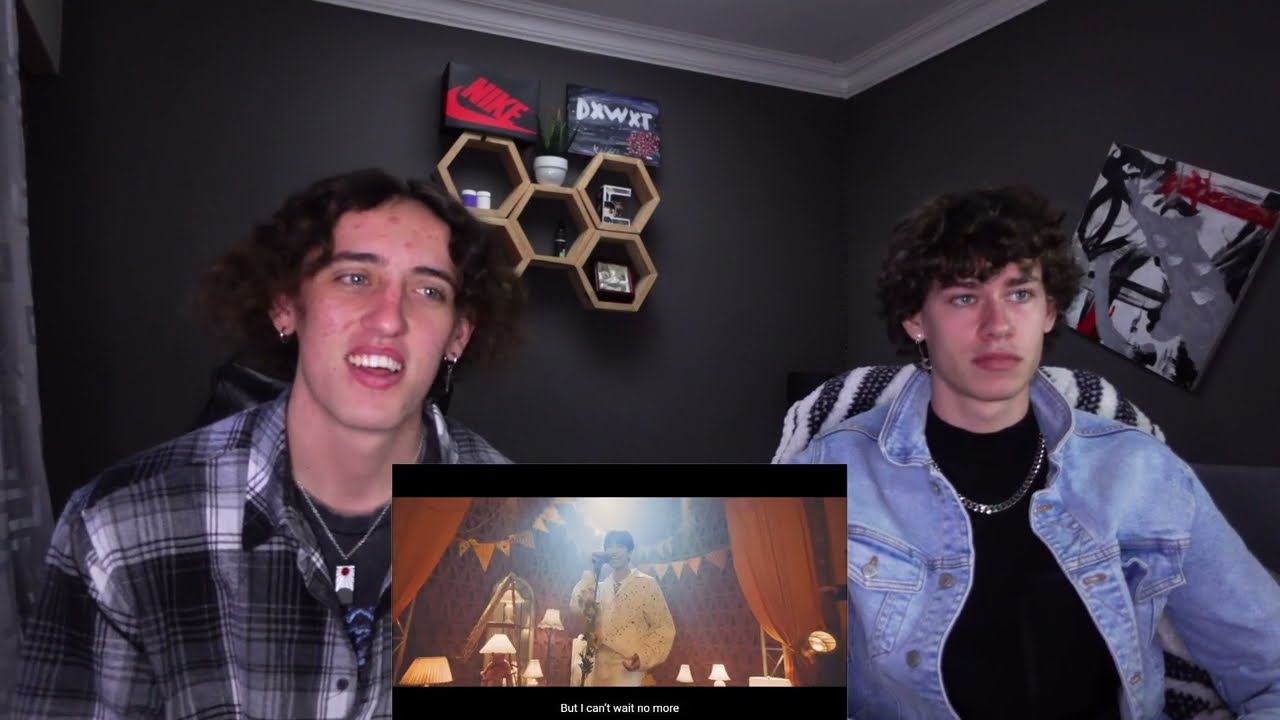This image captures two young Caucasian men, possibly in their late teens or early twenties, seated side by side in what appears to be a bedroom with dark gray walls and a white ceiling. Both have curly hair; the individual on the left sports a black and white plaid shirt over a gray tee, acne, and an earring, whereas the person on the right wears a jean jacket over a black shirt with a gold chain, and also has an earring.

They appear to be engaged in watching a video, likely a music performance given the presence of a screenshot centered at the bottom of the frame. This smaller video frame shows a singer on stage, surrounded by orange curtains and triangle flag banners, holding a microphone, dressed in a white outfit, with the words "but I can't wait no more" displayed in white text on a black background.

The background of the room features hexagonal, honeycomb-like shelves adorned with various items, including a small plant in a white bowl with green leaves. To the left, a black and red Nike shoebox can be seen, along with another black item labeled "DX W XT" in white letters. There's also abstract art comprised of white, black, red, and gray colors.

Overall, this scene exudes the typical setup of a reaction video commonly found on YouTube, where the two individuals provide commentary on the content they are watching.